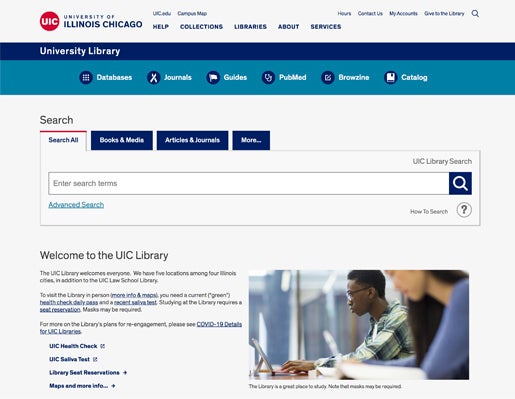This image is a screenshot of a University of Illinois Chicago (UIC) library website. The webpage background is an off-white color. 

At the top of the page is an off-white rectangle containing several navigation options. Starting from the left, there is a red circle with the text 'UIC' in white font. Next to this, in navy blue font, is the text 'University of Illinois Chicago.' Further along, it reads 'uc.edu, campus map, hours, contact us, my account, go to the library,' all separated by commas. Additionally, there is a magnifying glass icon representing the search function. Below these options are further links: 'help, collections, libraries, about, services.'

Beneath the off-white navigation bar, a navy blue banner displays the text 'University Library' in white. Under the navy banner lies a lighter blue rectangle featuring several options:

- 'Databases' represented by a navy blue circle with check marks,
- 'Journals' indicated by a navy blue circle with a twisted rope,
- 'Guides' symbolized by a navy blue circle with a flag,
- 'PubMed' denoted by a navy blue circle (the exact icon inside it is unclear),
- 'Browsing' shown by a navy blue circle with a white notebook and pencil icon.